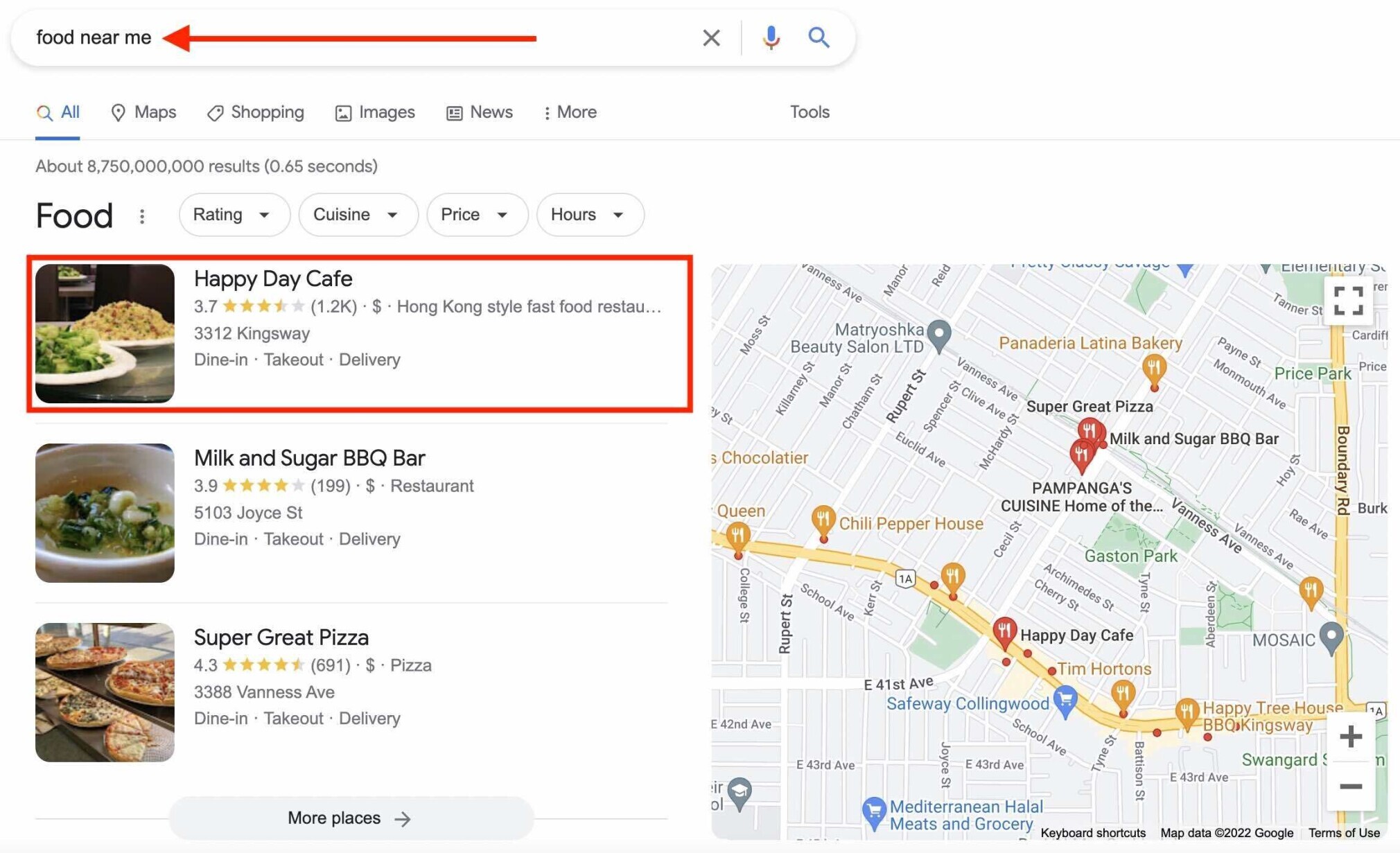Screenshot of a Google search results page for "food near me." The search options include tabs labeled "All," "Maps," "Shopping," "Images," "News," and "More," with a "Tools" button on the far right. Filters appear as bubbles with drop-down arrows for "Rating," "Cuisine," "Price," and "Hours."

To the right of the results, a map displays multiple food locations, with three spots highlighted. The first highlighted location is "Happy Day Cafe," marked in red, receiving 3.7 stars out of 5 from 1,200 reviews. It is a Hong Kong-style fast food restaurant, located at 3312 Kingsway, offering dine-in, take-out, and delivery options. The listing includes an image of two plates of food.

The second highlighted spot is "Milk and Sugar BBQ Bar," with a rating of 3.9 stars out of 5 based on 199 reviews. This restaurant is located at 5103 Joy Street and also offers dine-in, take-out, and delivery services. An image of a bowl of food accompanies the listing.

The third spot is "Super Great Pizza," boasting a 4.3-star rating out of 5 from 691 reviews. This pizza place is situated at 3388 Venice Avenue and provides dine-in, take-out, and delivery options. An image of a pizza pie is shown alongside the details.

A bubble indicating "More places" suggests additional locations not displayed in the initial screenshot.